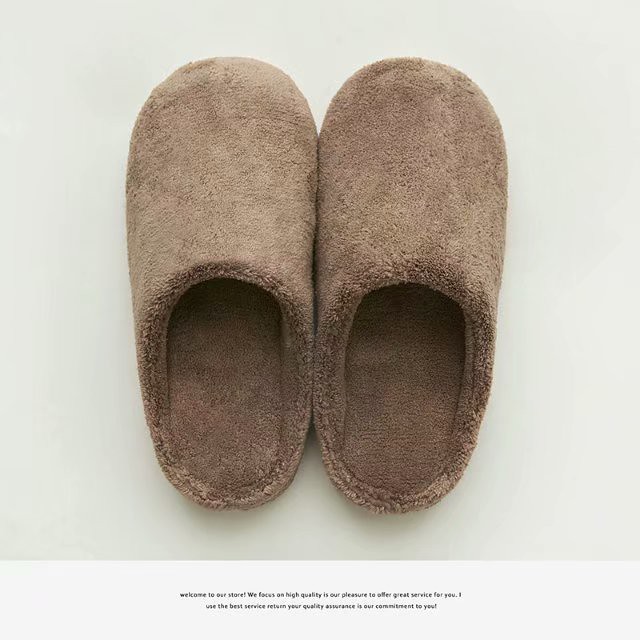This image is a detailed advertisement photograph showcasing a pair of light brown slippers with a quilted, fuzzy, terry cloth-like texture. These soft, insulated slippers, resembling penny loafers, feature perfectly rounded tops and flat soles, designed for maximum comfort and ease of use around the house. The slippers are positioned vertically in the center against a solid white gradient background, with shadowing highlighting the interior and brighter lighting on the top and toe areas. At the bottom of the image, a white strip contains small black text that reads, "Welcome to our store. We focus on high quality. It is our pleasure to offer great service for you. Use the best service return. Your quality assurance is our commitment to you." The text implies this is an advertisement from a retailer, possibly a smaller seller on a marketplace.